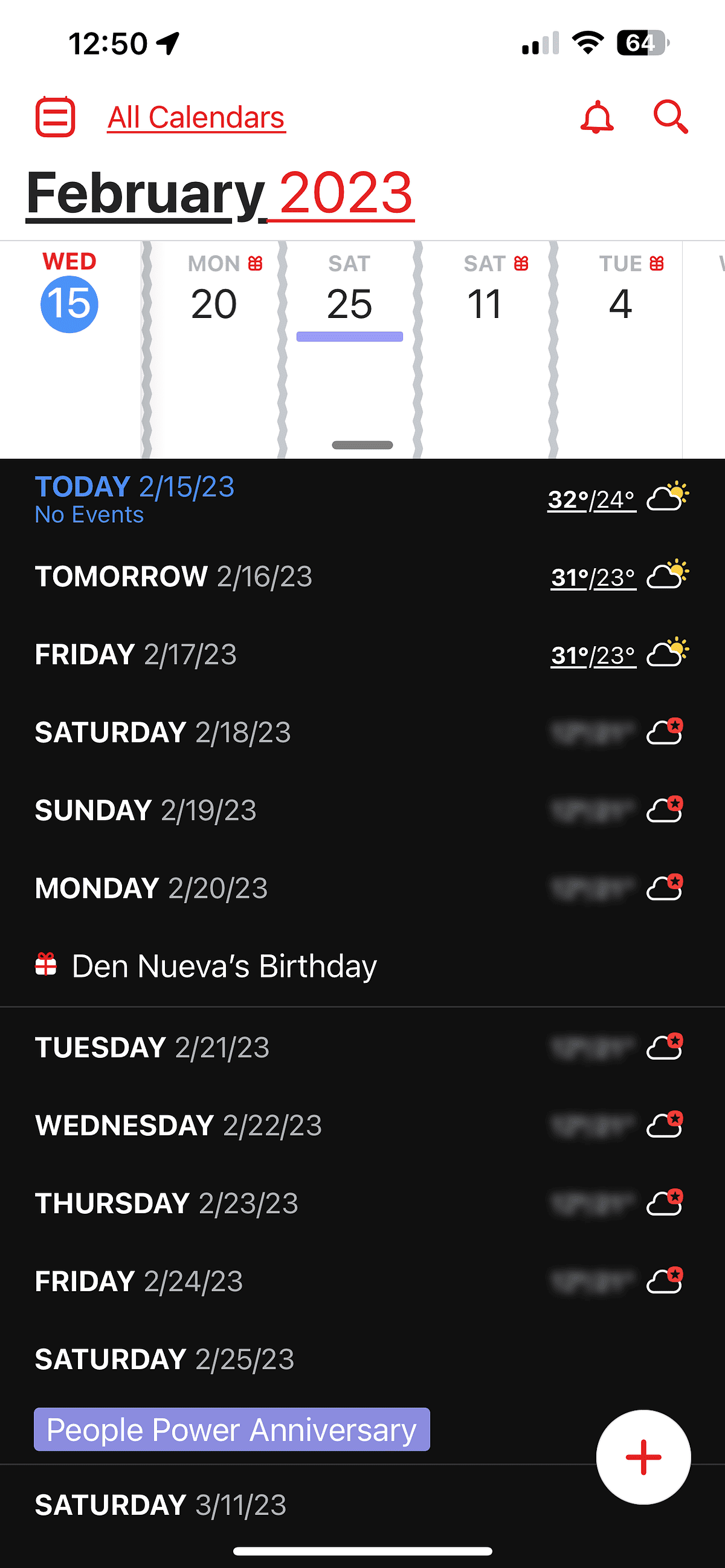The image appears to be a screenshot of a smartphone calendar app. The time displayed at the top-left corner is 12:50. To the right, there is a Wi-Fi signal icon and a battery icon indicating a 64% charge. At the upper left corner below the time, there is a red calendar icon next to the text "All calendars". To the right of these is a bell notification icon and a search icon.

Below this, the title reads "February" in black, followed by "2023" in red. Beneath the title, there is a list of days: Wednesday, Monday, Saturday, Saturday, and Tuesday with corresponding dates—Wednesday the 15th, Monday the 20th, Saturday the 25th, Saturday the 11th, and Tuesday the 4th.

A black rectangle labeled "Today, 2-15-23" indicates that there are no events scheduled for the current day. To the right of this, the weather forecast is shown, stating a high of 32°F and a low of 24°F with a partly cloudy icon.

Moving down the calendar, the dates continue sequentially: "Tomorrow, Friday the 1st," "Saturday the 18th," "Sunday the 19th," "Monday the 20th," followed by "Tuesday the 21st," "Wednesday the 22nd," "Thursday the 23rd," "Friday the 24th," and "Saturday the 25th." There is a pop-up notification mentioning "Den Nueva's birthday" with an image of a present. Another event listed in purple text indicates "People Power Anniversary" on Saturday the 11th.

Weather icons are displayed on the right side of each day in the calendar.